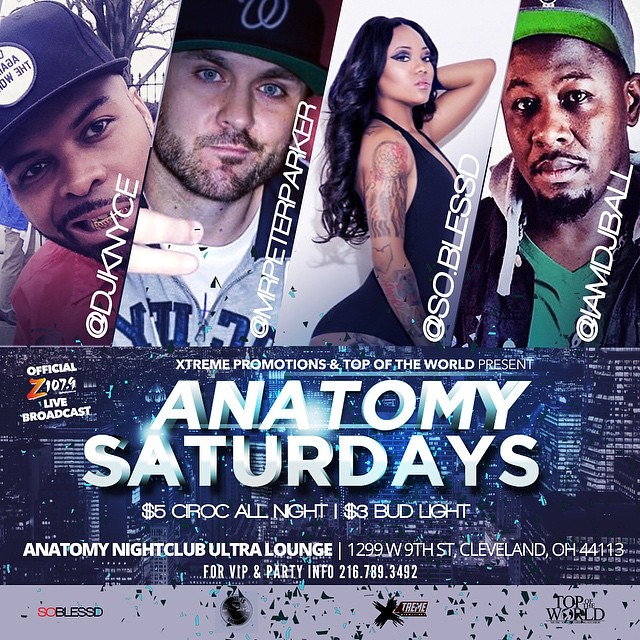This full-color poster for "Anatomy Saturdays" at the Ultra Lounge in Cleveland, Ohio, features four individual portraits of club artists, with city skyscrapers in the background. The images are arranged horizontally from left to right, starting with DJ K Nice, followed by Mr. Peter Parker, Esso Blessed, and I am DJ Ball. Each of the portrayed individuals—three men and one woman—has their name displayed in white lettering beneath their respective image. The men, two of whom are Black and one who is white, all sport facial hair and wear baseball caps, while the woman, who is also Black, has long black hair.

Below the photos, in bold capital letters, the text reads: "Anatomy Saturdays," presented by Extreme Promotions and Top of the World. This is followed by information about the event, including a $5 Ciroc all-night offer and $3 Bud Light. Additional details such as the club’s address, 1299 West 9th Street, Cleveland, Ohio 44113, and a contact number for VIP and party information (216-789-3492) are provided. Official Z107.9 live broadcast logos are also featured, emphasizing the event’s promotional sponsors.